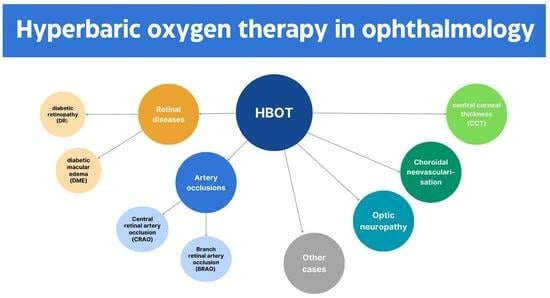The image is a horizontal, computer-generated color diagram focused on "Hyperbaric Oxygen Therapy in Ophthalmology" as highlighted in white text over a blue banner at the top. At the center of the diagram is a large blue circle labeled "HBOT." This central circle acts as a hub from which various colored circles radiate, each connected by lines indicating a relationship. Among these circles are terms such as "Artery Occlusions," "Retinal Diseases," "Optic Neuropathy," and "Choroidal Neovascularization." These primary circles further branch out into smaller circles, each detailing specific conditions related to their category. The intricate web of interconnected circles and lines visually maps out how various ophthalmic conditions are associated with hyperbaric oxygen therapy.